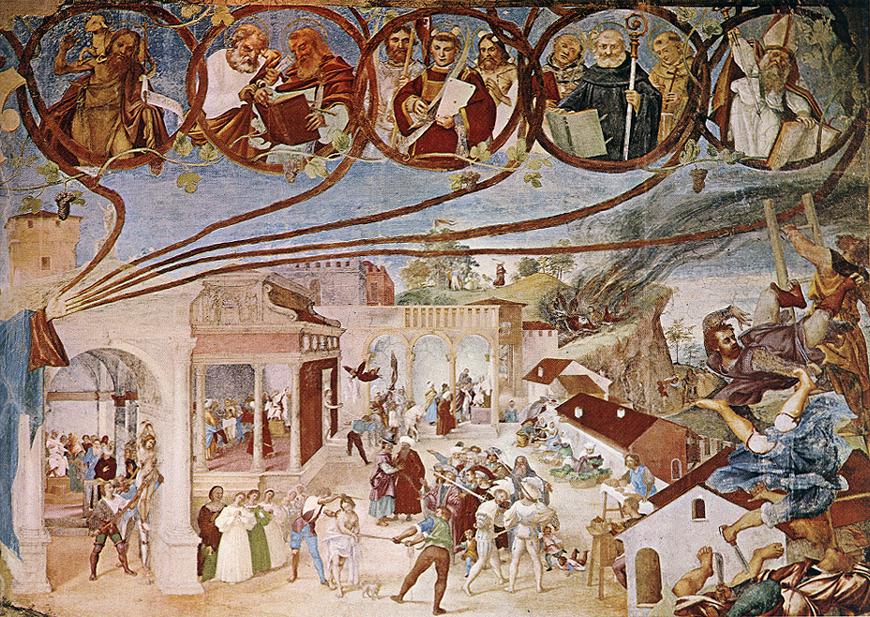This painting, possibly a mural from 17th-century Italy or Rome, depicts a richly detailed and intricate religious scene. At the focal point is a partially visible figure in a blue and red robe, extending an arm out of the cloak. Each of the figure’s fingers forms a line that culminates in five circles at the top of the painting, each containing distinct scenes.

- From the thumb, a line leads to a circle featuring a thin man and a white bird.
- The pointer finger's line reaches a circle with two bearded men reading a large brown book.
- The middle finger's circle contains three figures: two bearded men and a young boy holding a feather pen and paper.
- The ring finger connects to a circle where an old man in a black robe, holding a scepter, examines a large book flanked by two other figures.
- The pinky finger's circle portrays a man with a white beard, dressed in a white robe and pointed hat, wearing a red cape, clutching a book in one hand and raising the other in apparent anger.

Below this celestial scene, a bustling town center unfolds with numerous figures engaged in various activities. To the right, people stand on an elevated balcony. The background reveals green hills and, in the distant perspective, an individual in a red tunic and a fire emitting black smoke. Central to the earthly realm are groups of people—jousters, men in tights and tunics—interacting in what appears to be a marketplace or public space. Women sing in a choir, directed by another figure, and a woman, possibly a slave, is carried by someone nearby. The myriad elements of this artwork combine to create a vivid tableau rich with mythological and philosophical references, framed in a deeply religious context.